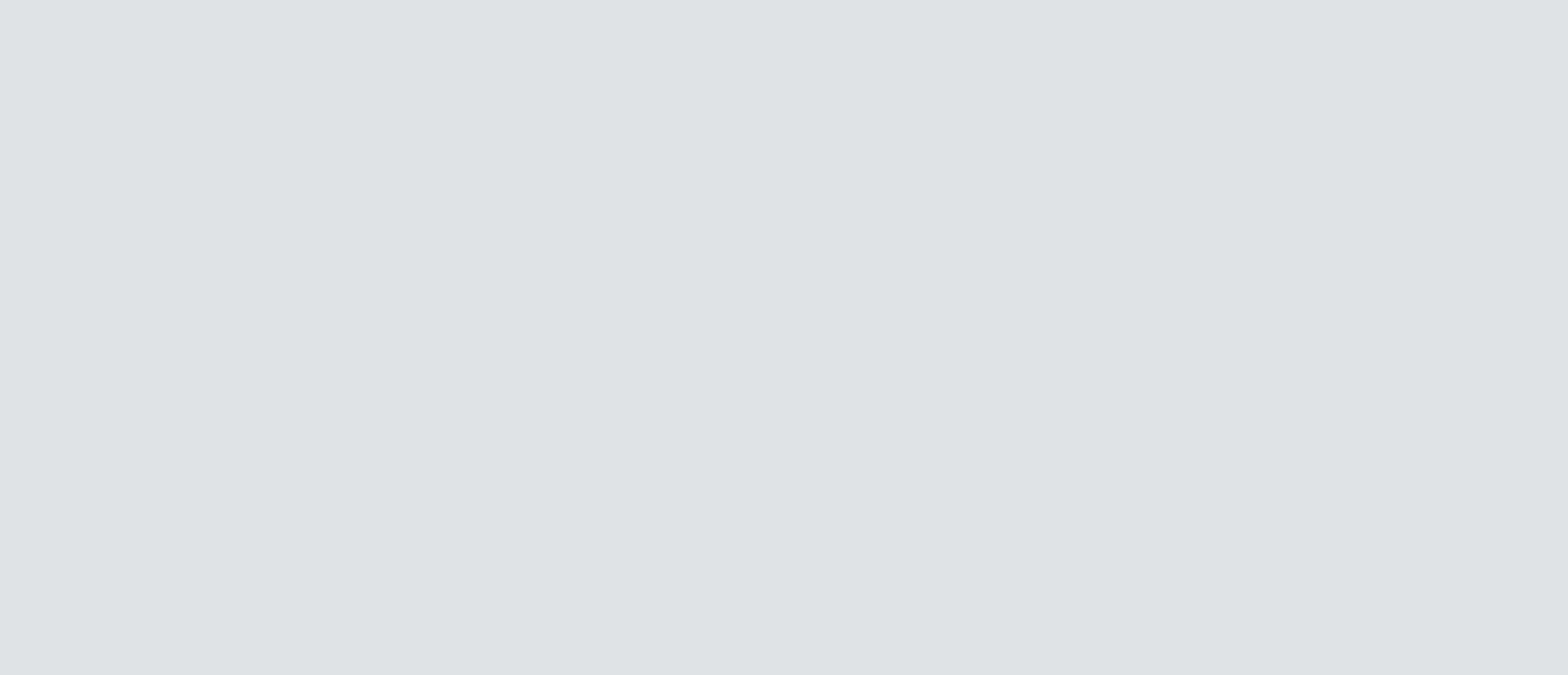The image features a landscape-oriented, perfectly rectangular gray box set against a stark white background. The box, approximately two to three times wider than it is tall, contains no text, images, or visible elements — it's entirely blank. This minimalist scene could either be a deliberate design choice or a result of a technical glitch, as it's unclear whether content was supposed to populate the center of the gray box. Its simplicity is perplexing, inviting speculation about what might have been intended for this space.